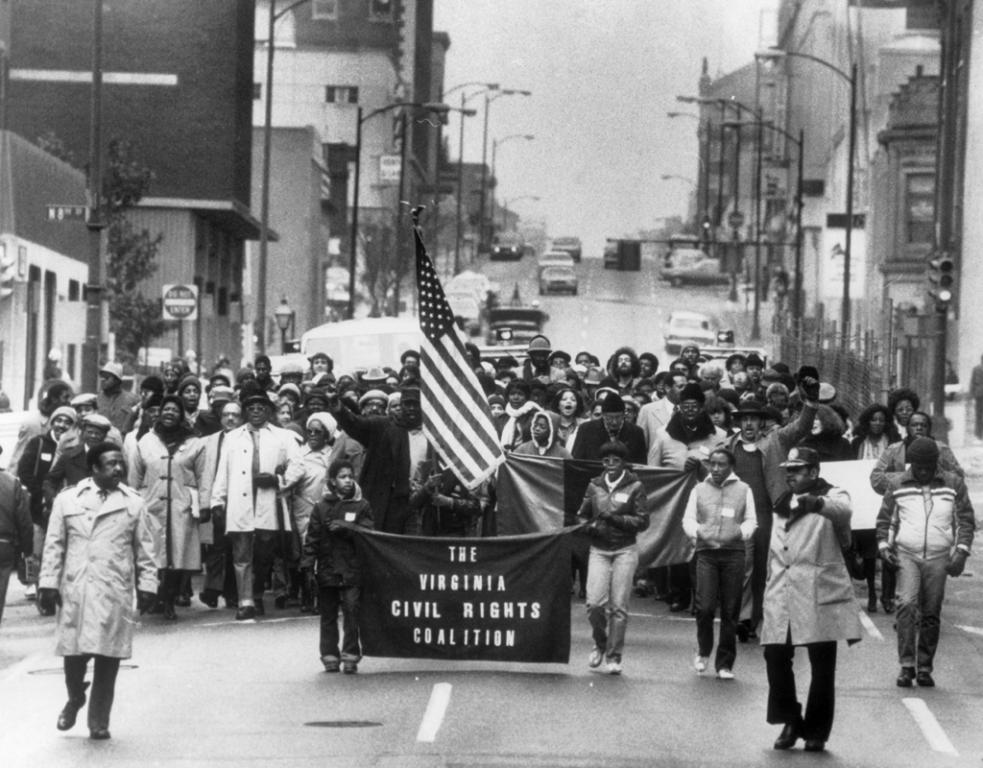This black-and-white photograph captures a historical civil rights march, likely taken in a major city during the late 1950s to mid-1960s. The scene is bustling with a crowd predominantly composed of African-American individuals, though there are a few Caucasians present as well. Central to the image are two African-American figures at the forefront— a woman on the right and a young boy on the left—holding a black banner that reads "Virginia Civil Rights Coalition" in white lettering. Both are dressed in winter attire, indicating the season. Flanking them on either side of the street are two men, also African-American, sporting long coats and black pants; the man on the left wears gloves, while the man on the right has a black baseball cap.

The marchers are proceeding down a slightly declining city street, which is lined with tall buildings and various street signs, including "Do Not Enter." In the background, cars are seen driving towards the gathered crowd. Adding to the visual impact, an American flag is prominently carried by participants further back in the procession, symbolizing their quest for equal rights. The overall atmosphere suggests a community united in solidarity for the cause of civil rights.